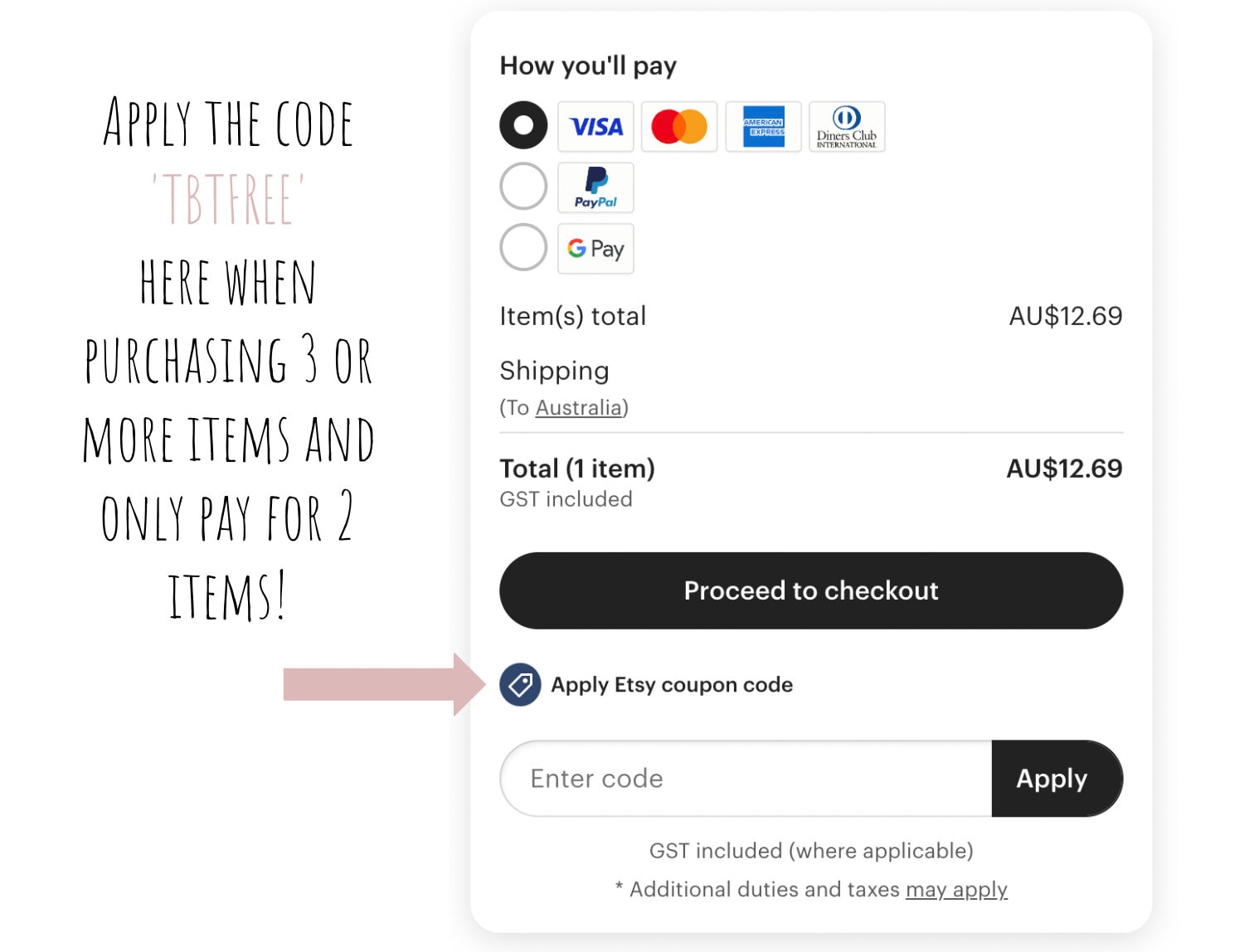**Detailed Checkout Screen Description:**

The image depicts a comprehensive checkout screen used for an online purchase, predominantly in shades of white, black, and light gray, with specific elements highlighted in other colors. 

Starting at the top left corner of the screen, the section reads "How you'll pay," followed by three payment options listed vertically: "by card," "by PayPal," and "by Google Pay." The "by card" option is pre-selected, and to the right of it, there are four payment card icons representing the acceptable card types.

Underneath the payment options is the order summary detailing the costs. The summary begins with "Item(s) total," which is listed as "AU $12.69" in parentheses. Below this, shipping information is provided: "Shipping to Australia," showing the destination and the total number of items, followed again by the cost of "AU $12.69."

Proceeding further down, there is a prominent, wide, black oval-shaped button labeled "Proceed to checkout" in white text, centrally located within the button.

Below the checkout button, there is a section inviting users to apply a discount code. Instructions are provided in gray text, which reads: “Apply the code 'TBT3' when purchasing three or more items and only pay for two items.” Directly beneath this is a light purple arrow pointing towards the section to apply the Etsy coupon code. 

Continuing downwards, users can enter their coupon code into a designated box and click "Apply," which is a button with a black background and white text positioned to the right of the entry field. 

Additional statements follow regarding applicable taxes and fees: "GST included (where applicable)" and "Additional duties and taxes may apply." The entire checkout area is set against a white background, while the outer frame of the screen is a light gray color, adding a clean and structured aesthetic to the interface.